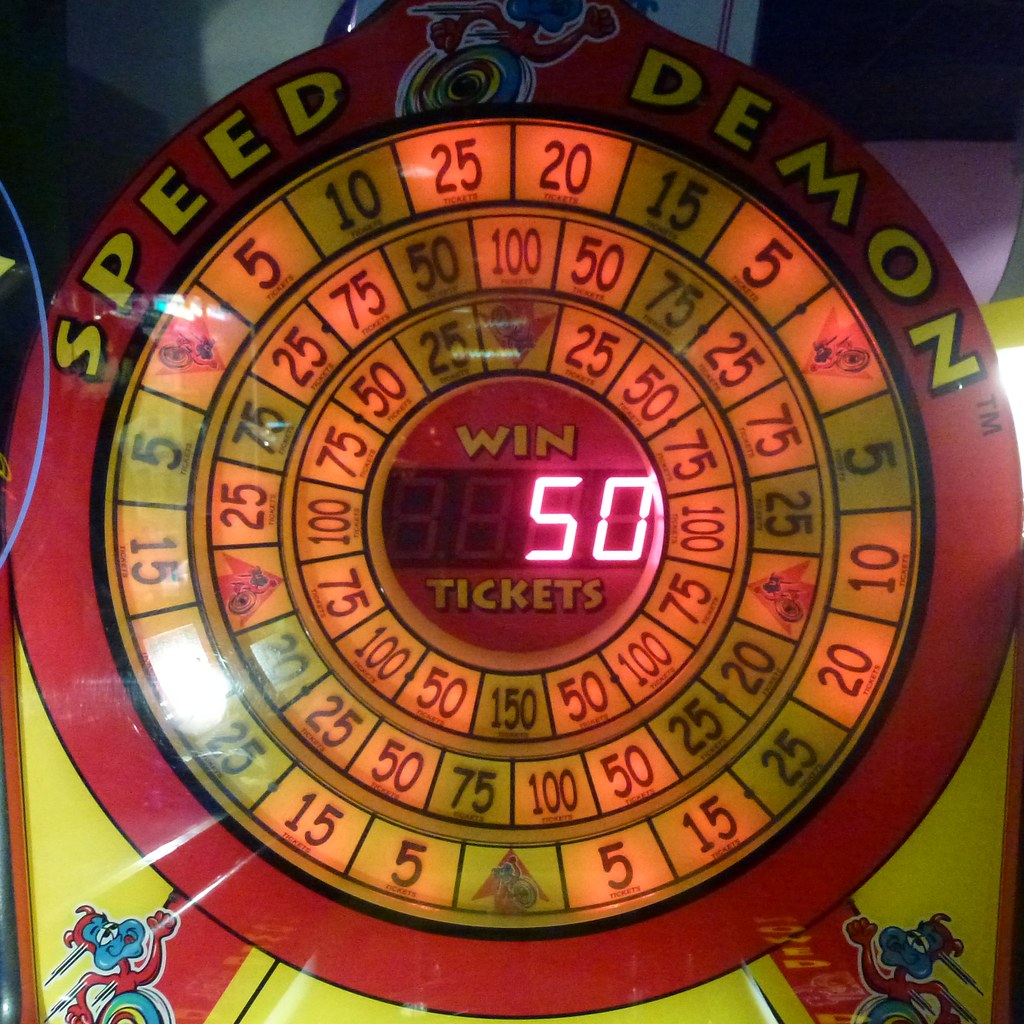This color photograph is a close-up of an electronic game called "Speed Demon" found in a game room. The game features a large circular wheel with the outermost red ring displaying the game's name, "Speed Demon," in yellow letters. Between the words "Speed" and "Demon," a small blue cartoon demon with red horns and red arms appears. Similar cartoon demons are located at the bottom corners of the image.

Inside the outer ring, there are three concentric rings with various numbers, representing ticket amounts that can be won. These numbers include, but are not limited to, 5, 10, 15, 20, 25, 50, 75, and 100, displayed in red lettering. Some of these numbers are illuminated. At the very center of the wheel, in a red and yellow section, the words "Win Tickets" are prominently featured. Directly below this, a digital display shows the number 50, indicating the player has won 50 tickets. Each ring is filled with lit-up ticket values, contributing to the game's dynamic appearance.